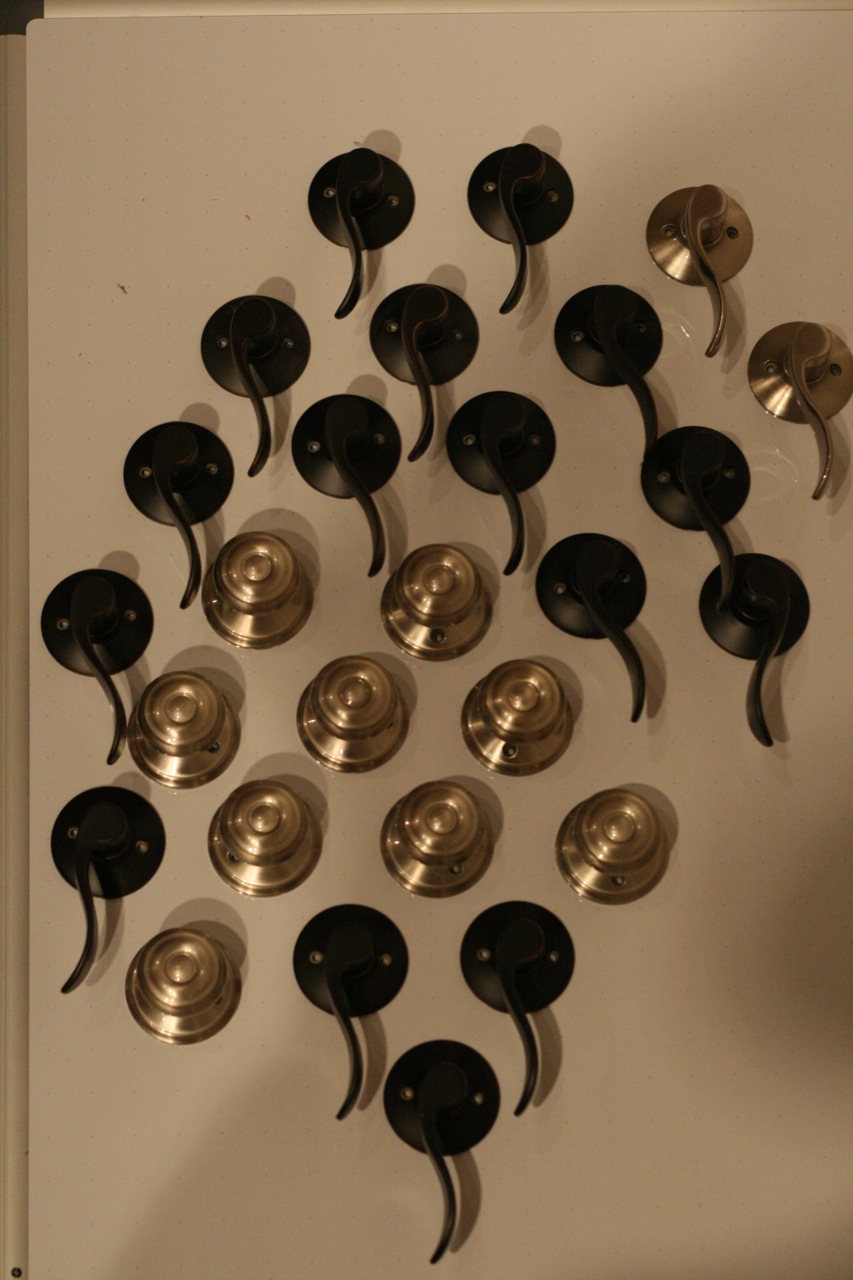The photograph displays an array of doorknobs and door handles on a flat, dingy-looking beige surface, captured in portrait orientation from an overhead angle. The lighting in the image is poor, casting the scene in shadows. The surface is cluttered with doorknobs and handles, which are made of metal. There are a total of 27 objects scattered randomly: 11 are a silver color and 16 are black. The handles have a round piece with a thin, curved handle. Some of the doorknobs are described as golden or brown, featuring grooves and the typical button found on interior door knobs. The black handles are characterized by their long, arching pulls. The arrangement appears to lack a discernible pattern, contributing to a disorganized presentation.